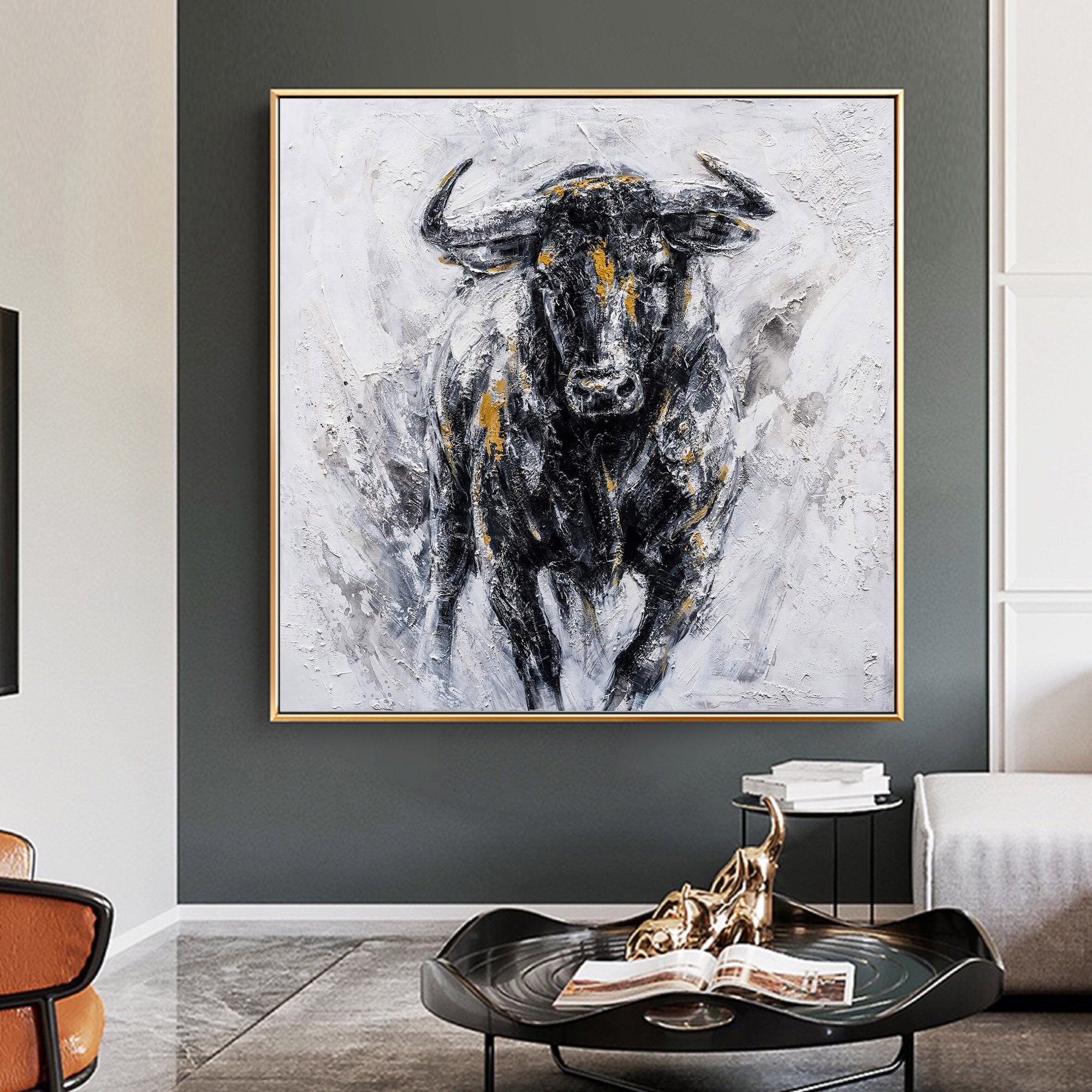The photograph captures a living room dominated by a striking piece of artwork. The main attraction is a large, square painting almost covering a greenish-gray wall. Encased in a thin gold frame, the artwork depicts a black buffalo accented with streaks of brown and gold, rendered with a blurred, non-linear style. Below the painting, a low, black coffee table sits centrally, holding an open book and a gold figurine. To the right, a small round-topped table supports three books, accompanied by a white ottoman. The floor features gray, marble-like tiles. Additionally, in the lower left-hand corner, a hint of an orange and black chair is visible, adding a touch of contrasting color to the setting. The room's design brings a harmonious blend of modern and rustic elements.